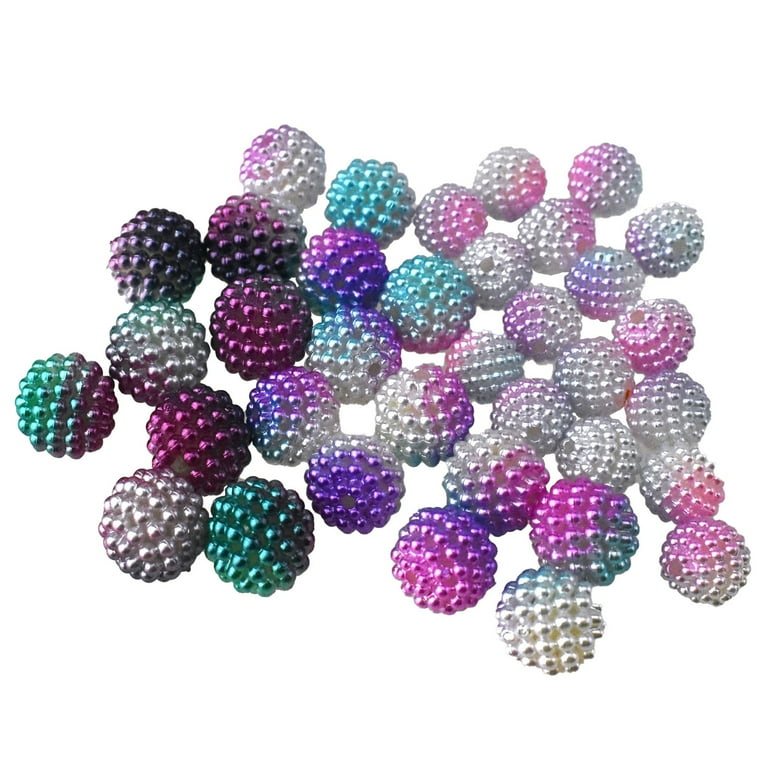This image portrays a mesmerizing close-up of approximately 40 intricately textured beads resembling clusters of berries, each adorned with small ridges similar to those on blackberries or raspberries. The beads are a beautiful assortment of colors, including various shades of greens, purples, silvers, teal, magenta, and white, creating a vibrant and dynamic visual. They exhibit an ombre effect, where one bead blends from one color to another, adding to their pearlescent and multifaceted appearance. Light appears to be streaming in from behind, enhancing their gleam and making them look exceptionally shiny and radiant. The arrangement suggests a gradient from darker hues on the left side to lighter, more pearlescent tones on the right. Some beads also display small holes, hinting at their potential use in crafting. Altogether, the image creates a striking and colorful spectacle, with the beads jumbled together in a captivating pile.